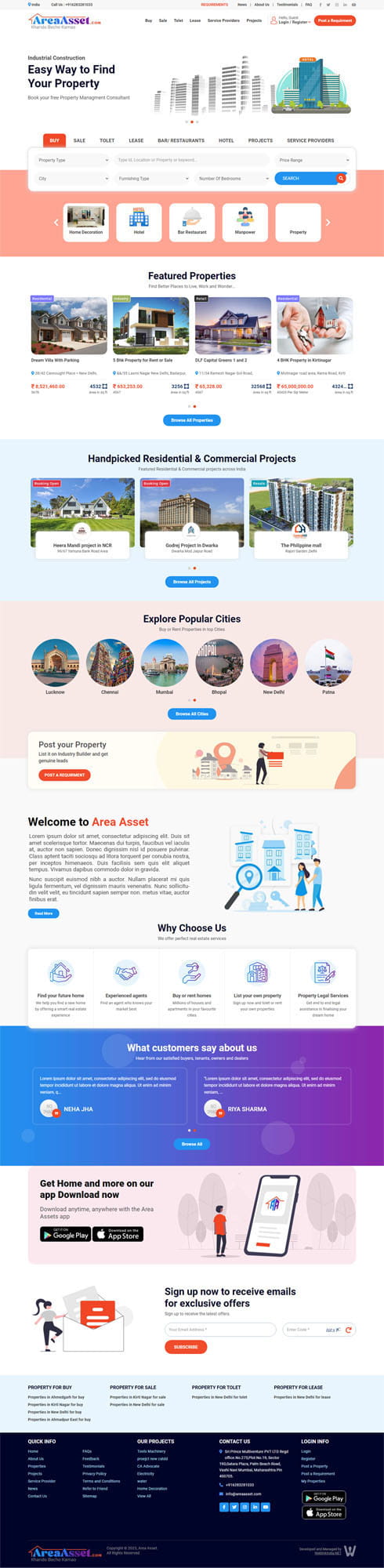This thin rectangular image, oriented vertically, showcases a website interface, likely related to real estate or rental services, potentially reminiscent of a platform like Airbnb. At the very top, a gray border spans the width of the image, containing text that is too small to decipher. Directly below this top border, another header section features a horizontal menu bar. Within this header, an orange box with white text is situated on the right side, accompanied by an image of a city landscape.

Progressing downward, a second horizontal menu is present, with the leftmost option highlighted in orange, suggesting it is the current selection. Below this, there is an orange box interspersed with white boxes bearing various symbols. Towards the center of the image, the text "Easy way to find your property" is legible, hinting at the site's purpose as a real estate or rental search platform.

Further down, a segment labeled "Featured Properties" displays three images of different homes or properties. An additional image showcases a hand holding a set of keys. At the bottom of the image, a blue box with white text can be observed. The overall interface features a blend of multiple colors, boxes, and images, contributing to a visually organized layout for browsing properties.